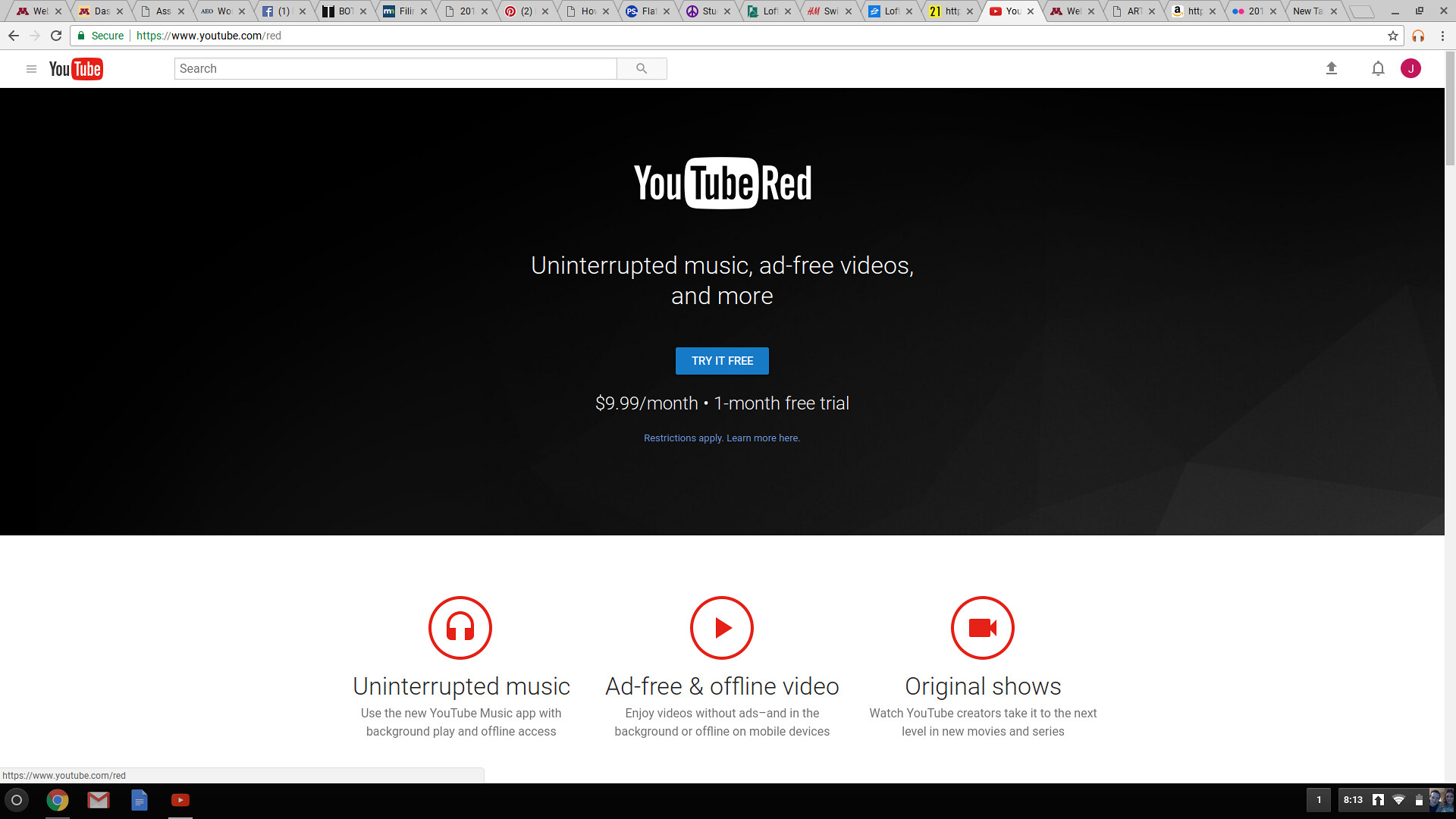A screenshot of a personal computer is displayed in the image. The screen is in landscape mode, featuring a long, narrow rectangular shape. At the top of the screen, a plethora of tabs are open—easily over a dozen. The screenshot is focused on a YouTube Red promotional page, which occupies the majority of the visible screen.

In the upper left corner, the familiar YouTube logo is displayed. The main section of the screen is predominantly black, showcasing the YouTube Red branding in bold white letters. Below this, a tagline reads: "Uninterrupted music, ad-free videos, and more." Further down, a blue rectangular button featuring white text invites users to "Try it free." Adjacent to this button, another text segment states: "$9.99 per month, one month free trial."

Lower on the page, a contrasting white section appears, highlighting three distinct features of YouTube Red. On the left, a red circle with a headphones icon promotes "Uninterrupted music," accompanied by additional details. In the center, a red circle with a right-pointing arrow symbolizes "Ad-free and offline video." To the right, a red circle with a movie camera icon signifies "Original shows."

Along the bottom edge of the screen, a black border hosts small icons, including the Google Chrome icon, an email icon, and several others that are too small to identify clearly.

The image captures a detailed view of the promotional elements for YouTube Red, showcasing the service's key features and subscription details.